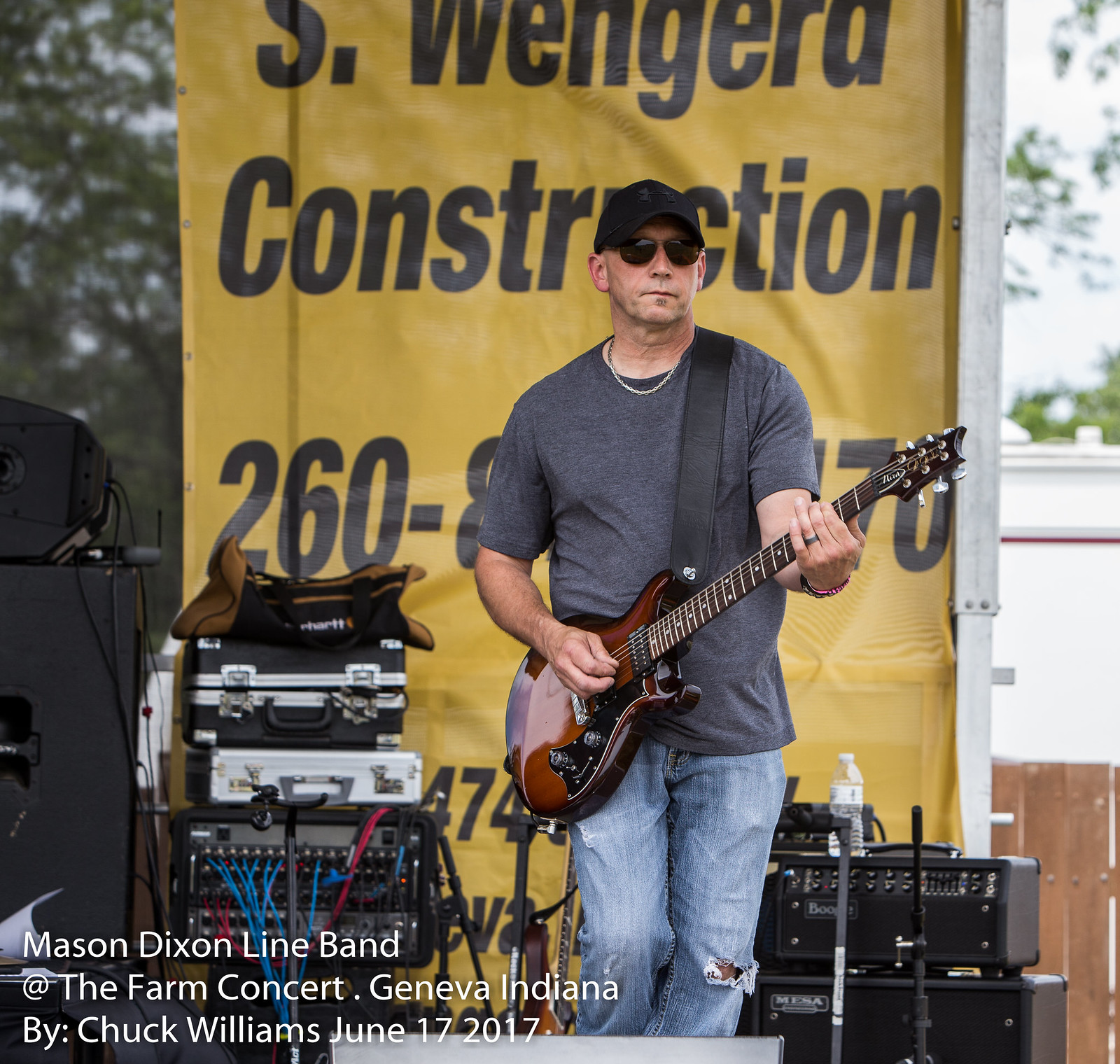The photo captures an outdoor music concert featuring a man with a serious expression playing an electric guitar in a performance setting. He is dressed in a black baseball cap, dark sunglasses, a gray sweatshirt, and distressed jeans with a hole on one knee. He also wears a silver necklace. The guitar he is playing is a shiny sunburst brown and black color, hanging from a strap around his shoulder as he stands with slightly bent knees. Behind him, there is an assortment of sound equipment, cables with blue and red wires, and speakers. A yellow banner with black text reading "S. Wengerd Construction" hangs in the background. The scene is set outdoors with trees and a bright overcast sky visible beyond the stage. At the bottom of the image, a caption reads, "Mason Dixon Line Band at the Farm Concert, Geneva, Indiana by Chuck Williams, June 17, 2017."